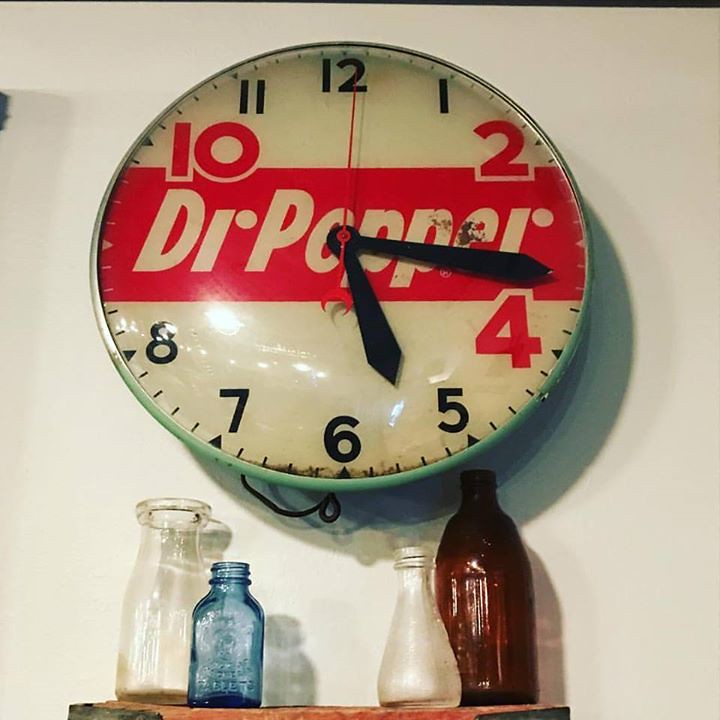In this photograph, we are presented with a dimly lit room, providing a nostalgic and slightly shadowed ambiance. The focal point of the image is a vintage round clock mounted on the wall. The clock's exterior is light green, encasing an antiqued cream face that shows signs of rust and wear, enhancing its vintage charm. Prominently displayed on the clock face amid a red stripe is the logo "D. Dr. Pepper." The numbers on the clock are a mix of red and black, with the 10, 2, and 4 o'clock positions distinctly marked in red.

Below the clock, a small wooden shelf is affixed to the wall, holding a collection of four glass bottles, each unique in design and color. From left to right, there is a clear bottle resembling an old-fashioned milk bottle, next to it a smaller blue glass bottle, followed by a white, genie-shaped bottle, and lastly, a larger brown bottle. The arrangement of these vintage bottles adds to the nostalgic atmosphere of the setting, creating a charming and timeless vignette.